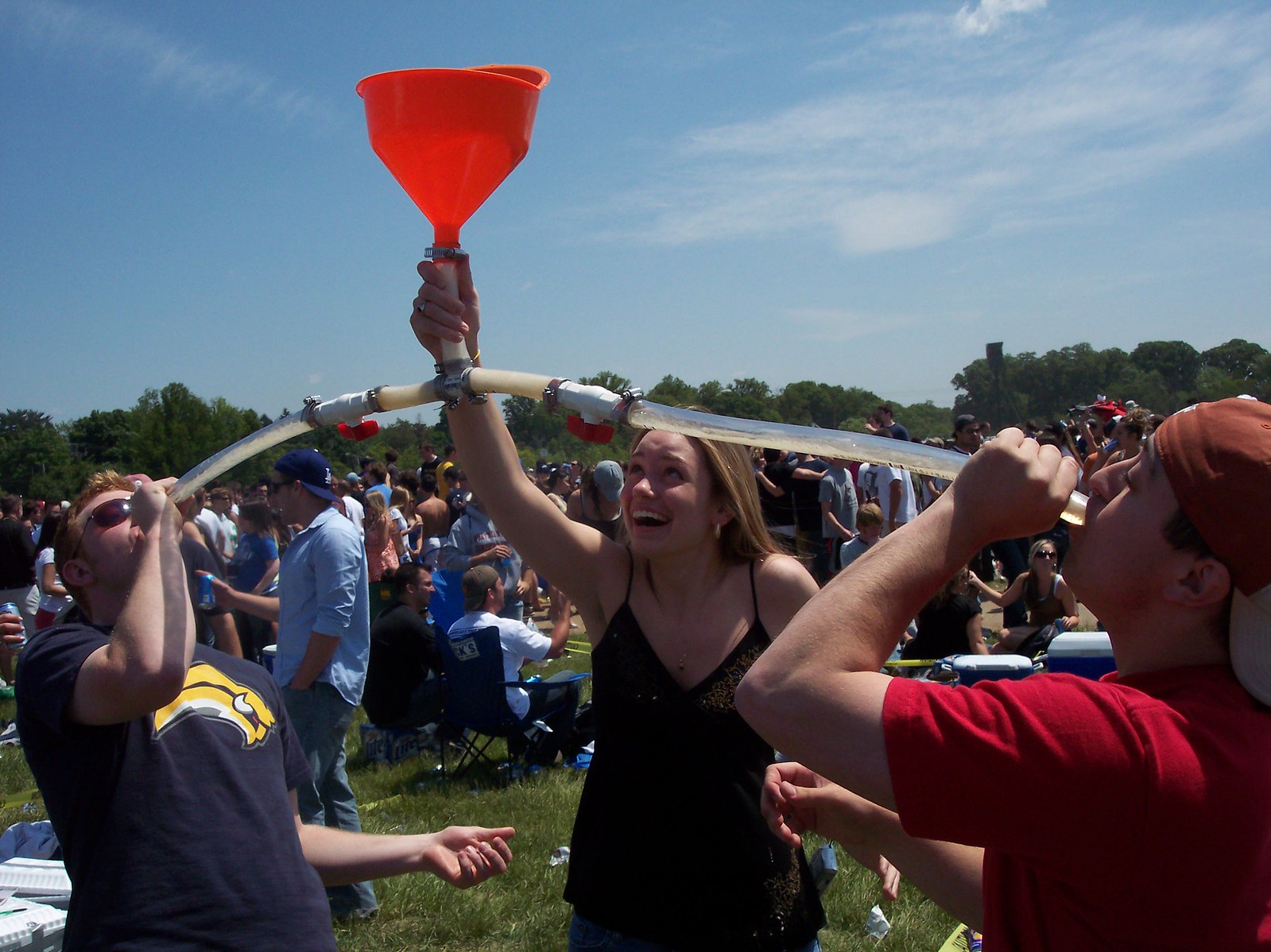In a vibrant outdoor gathering set in a sprawling grassy field, a young woman with light brown hair, dressed in a spaghetti strap black top and blue jeans, stands at the forefront holding a red beer funnel high in the air. This funnel divides into two long tubes extending towards two young men on either side. The man on the left, sporting a navy blue shirt emblazoned with a yellow bison and wearing sunglasses, leans back to chug beer from his tube. The man on the right, in a red shirt and a backward brown hat, mirrors this action with his own tube. This lively scene is bathed in the light of a bright blue sky, nearly devoid of clouds, with a crisp tree line of dark and light green foliage in the distance. The field is buzzing with numerous people, some seated in fold-out patio and butterfly chairs, mingling around coolers, all contributing to the festive atmosphere.